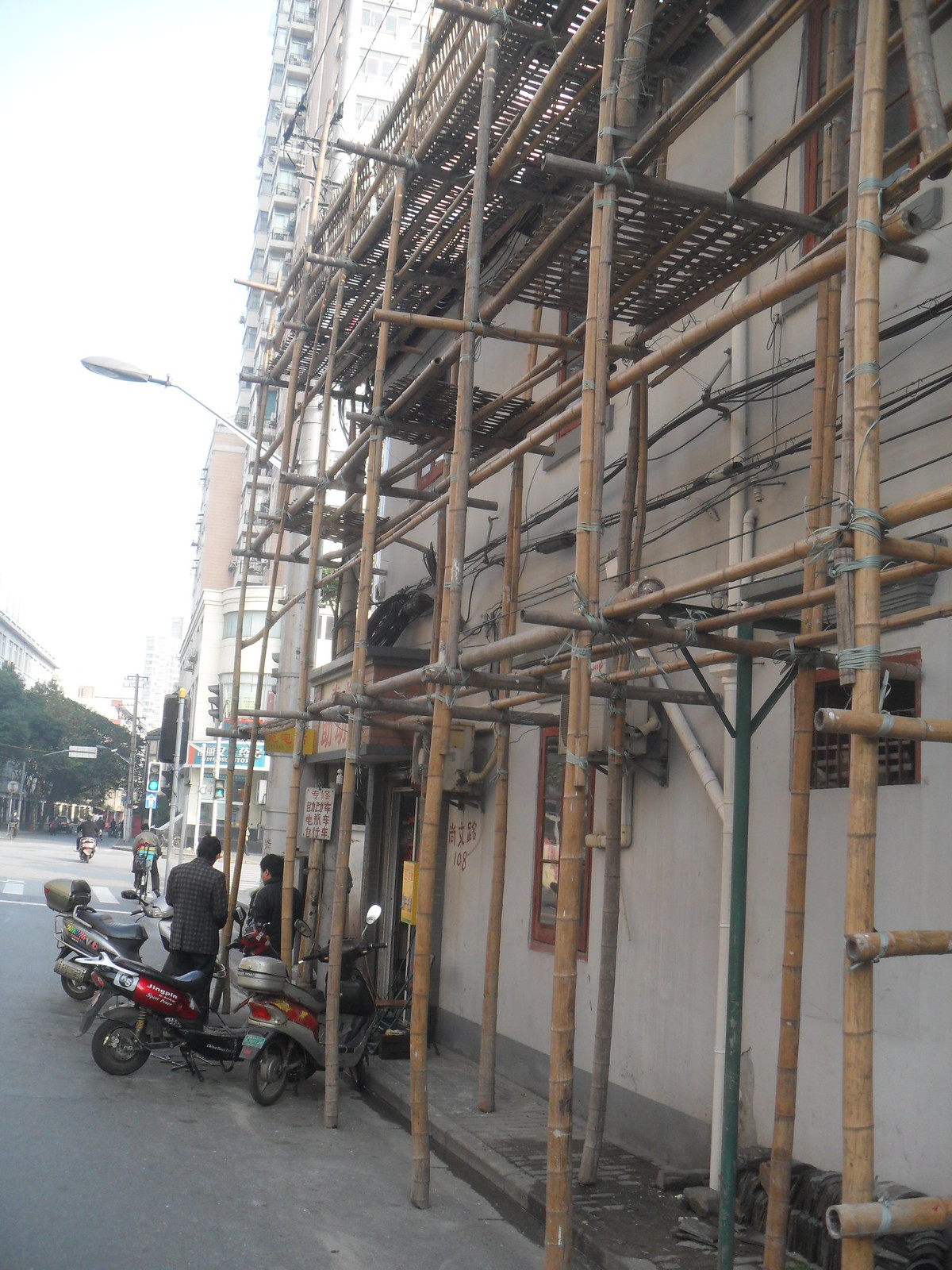The image captures a bustling street scene in what appears to be an Asian city, indicated by signs in Chinese text. The central focus is a building undergoing construction or renovation, supported by an intricate bamboo scaffolding structure that climbs the side of the white or beige wall. The scaffolding appears to be multi-leveled, providing pathways for workers to navigate and work on the siding. Below, two men stand near several parked red scooters, engaged in conversation. One man is dressed in a gray suit jacket, adding a touch of formality to the otherwise industrious setting. Surrounding the main scene, additional buildings can be seen in the background along with greenery from nearby trees. Street lights and other mopeds further populate the scene, adding to the urban atmosphere.